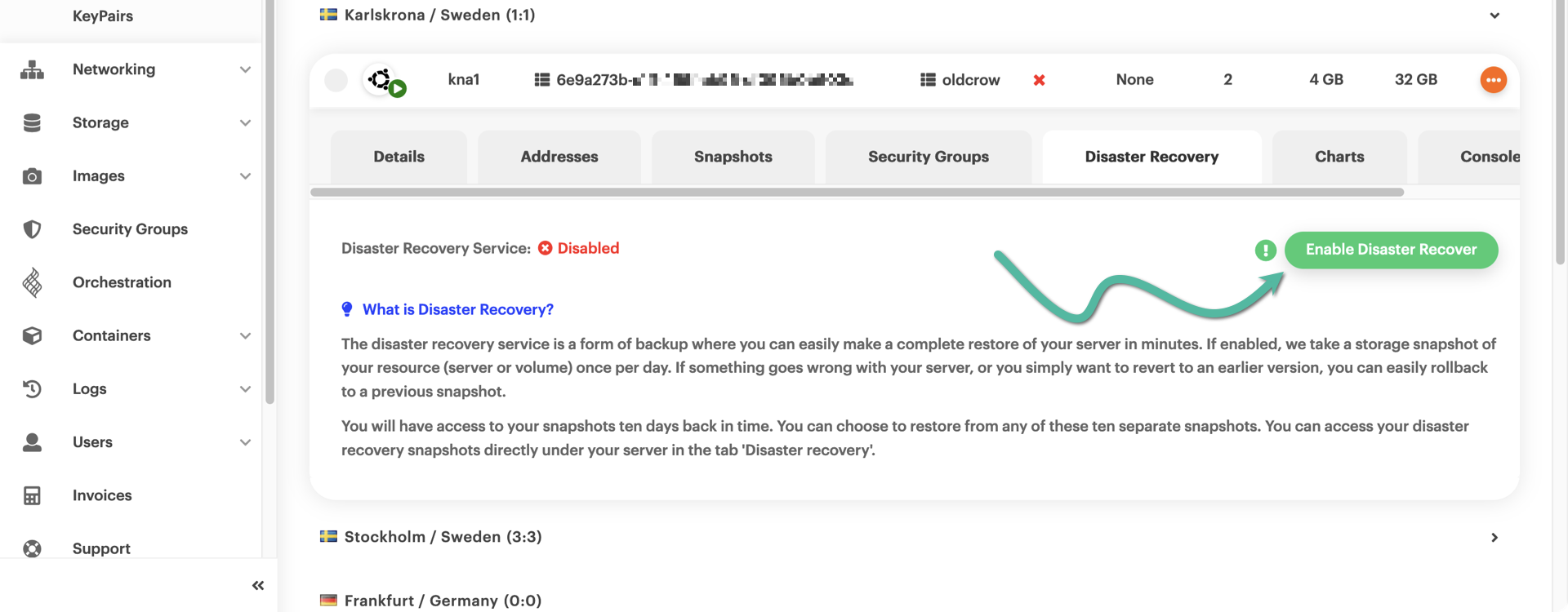The image appears to be a screenshot of a computer interface displaying various options and categories related to cloud management. On the left side of the screen, a vertical menu is visible, listing categories such as "Key Pairs," "Networking," "Storage," "Images," "Security Groups," "Orchestration," "Containers," "Logs," "Users," "Invoices," and "Support." 

To the right of this menu, at the top of the screen, the text "KARLSKRONA, Sweden" is prominently displayed, followed by "(1, 1)" in parentheses. Beneath this, the search bar shows the term "KNET" with horizontal options like "Details," "Addresses," "Snapshots," "Security Groups," "Disaster Recovery," and "Charts."

A green squiggly line with an arrow points towards a green box which contains the text "Enable Disaster Recovery." Below this, in blue text, a link labeled "What is Disaster Recovery?" is followed by an informational section enclosed in quotations. This section explains that users will have access to their snapshots for up to ten days and can choose to restore from any of these snapshots. It also mentions that disaster recovery snapshots can be accessed directly under the server in the "Disaster Recovery" tab.